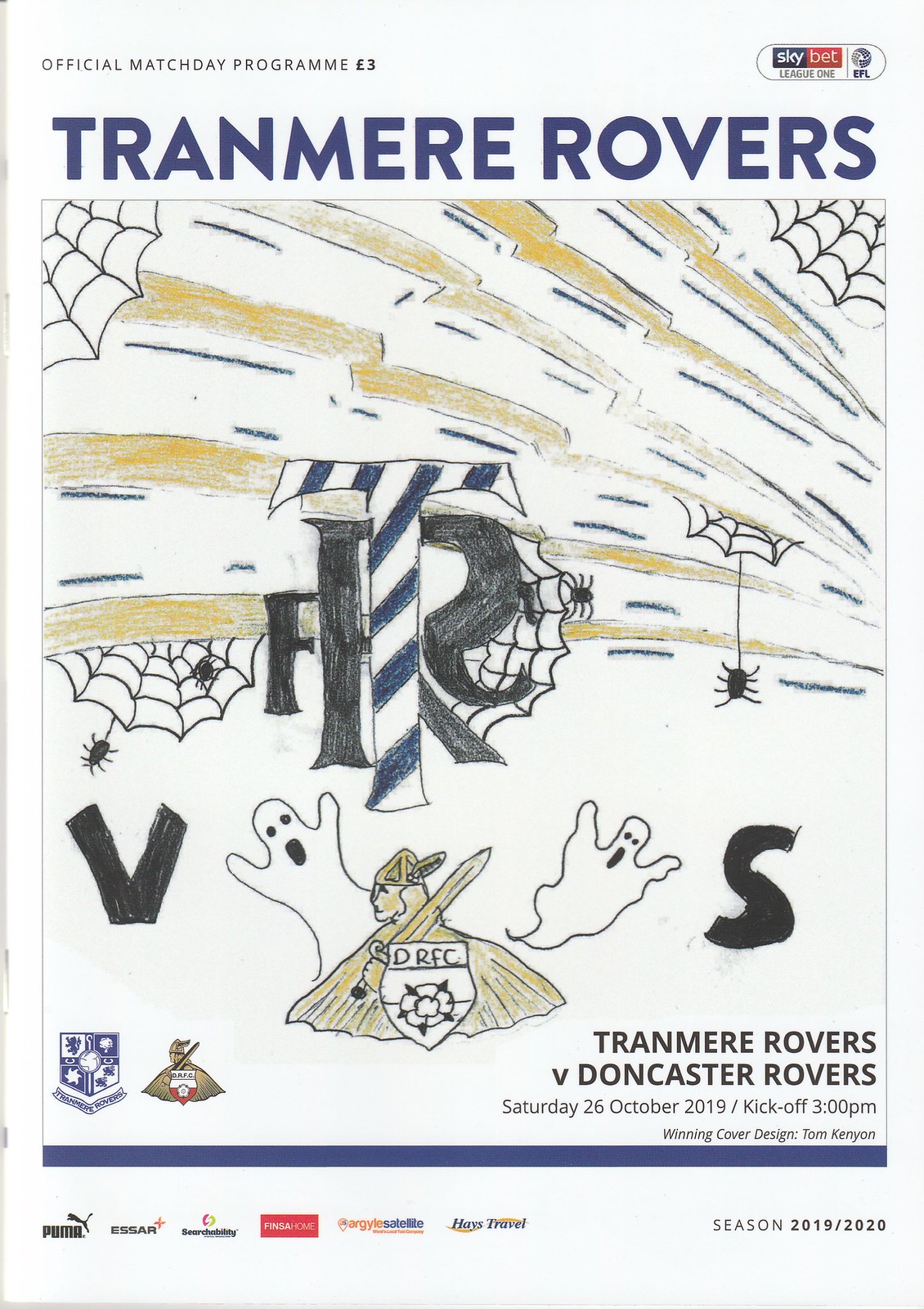This image appears to be the cover of an official match day program for a British football (soccer) game, specifically for a Sky Bet League One match. The program is priced at three pounds and prominently features text in the top left corner stating "Official Match Day Program" and the league designation in the top right corner. The main title, "Tranmere Rovers," is boldly displayed at the top center.

The centerpiece of the cover is a hand-drawn, childlike illustration, possibly created by a fan contest winner. The artwork has a Halloween theme with multiple spider webs and spiders, along with lightning bolts streaking across the sky. The illustration also includes two ghosts emerging from the ground.

Central to the drawing is a large 'T' superimposed over an 'R,' surrounded by more letters. There is also a depiction of the Doncaster Rovers logo, featuring a Viking-like figure holding a shield with the initials 'DRFC.' 

At the bottom, details of the match are listed: "Tranmere Rovers v Doncaster Rovers, Saturday, 26 October 2019, kickoff 3pm." The cover design is credited to Tom Kenyon for the 2019/2020 season.